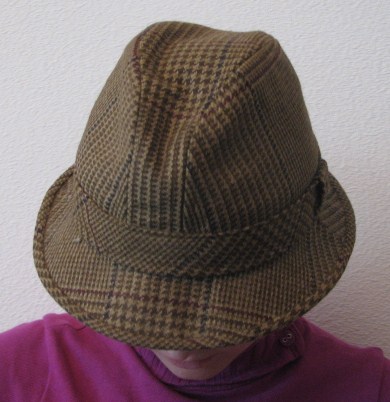The image depicts a light-skinned individual whose gender is not easily discernible due to the limited visible facial features—their nose, lips, and chin. They are looking down, obscuring their eyes. The person is adorned with a prominent hat, described variously as a brown hat with a design, akin to a fedora with green, red, and black stripes. The headwear evokes a stylish, almost Sherlock Holmes-like aesthetic. They are dressed in a purplish shirt or a thick sweatshirt with a distinctive collar resembling a zip-down turtleneck. Additionally, a button is visible on one shoulder. The backdrop is a white, textured wall, and the individual occupies most of the frame.